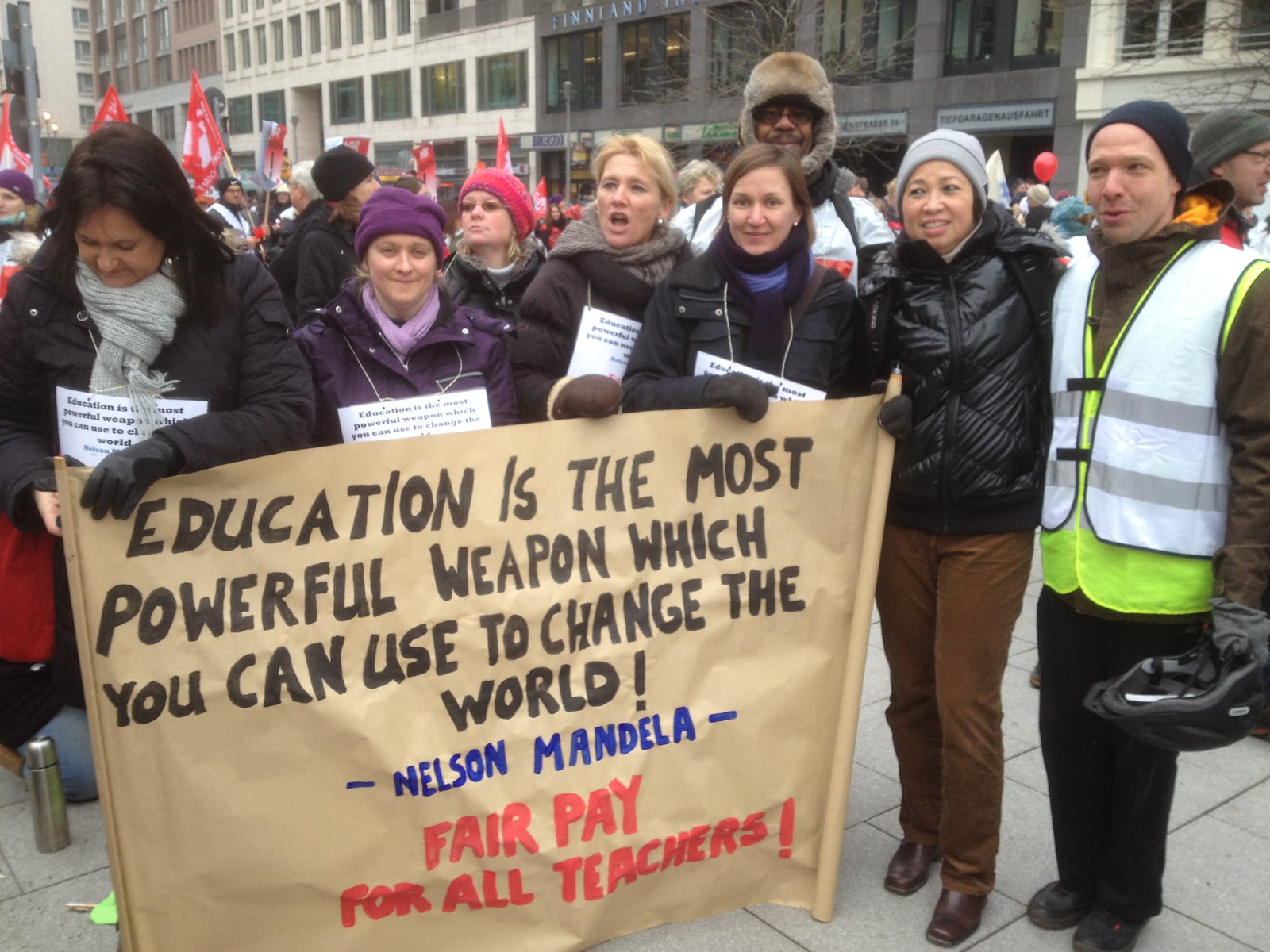This wide rectangular photograph captures a bustling city protest, with tall buildings and a busy urban street as the backdrop. The crowd, bundled up in puffy jackets, hats, and scarves against the cold, occupies a sidewalk paved with gray tiles. In the foreground, four women on the left side of the image hold a somewhat rolled-up, crinkled gray sign. The sign's top section features black, italicized, all-capital letters reading, "EDUCATION IS THE MOST POWERFUL WEAPON WHICH YOU CAN USE TO CHANGE THE WORLD." Beneath, in bright dark blue letters, it attributes the quote to "Nelson Mandela." The bottom section of the sign, in conspicuous bright red letters, demands "FAIR PAY FOR ALL TEACHERS!" The scene suggests the teachers are striking, unified in their call for higher pay, and are joined by others in the background, some of whom are holding flags and appear to be part of the larger rally. The surrounding skyscrapers with their myriad windows amplify the sense of an organized, significant city protest.